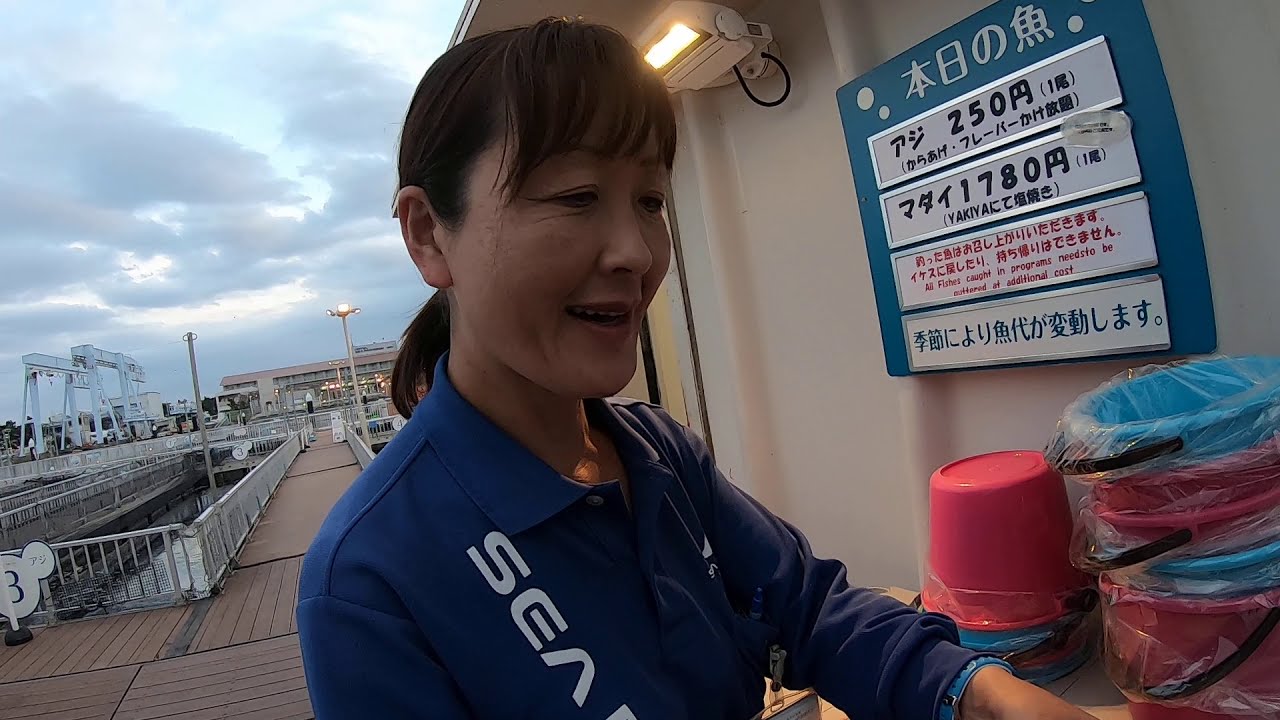The photograph captures a detailed outdoor scene of an Asian woman, likely in her late 40s or early 50s, with dark brown hair tied back in a ponytail and bangs. She is seen from her mid-chest up to the top of her head, standing at a countertop. The woman is wearing a long-sleeve blue collared shirt with white writing that partly reads "C something" and a light blue watch. She is faced three-quarters towards the right side of the image and appears to be looking downward.

The setting is a pier-like wooden walkway with white fencing around it, leading to other walkways over a body of water. The background reveals a white vinyl building to her right, which has a blue sign with white Asian characters and several smaller signs in different colors—black, red, and blue. There are also plastic buckets in an assortment of colors (red and aqua blue) with black handles and lined with plastic bags on the countertop beside her.

Above her, the building has a beige-colored wall and a light fixture. In the distance, one can see additional brown buildings and a couple of grayish metal structures. The sky is predominantly gray with clouds, allowing minimal blue sky to peek through.